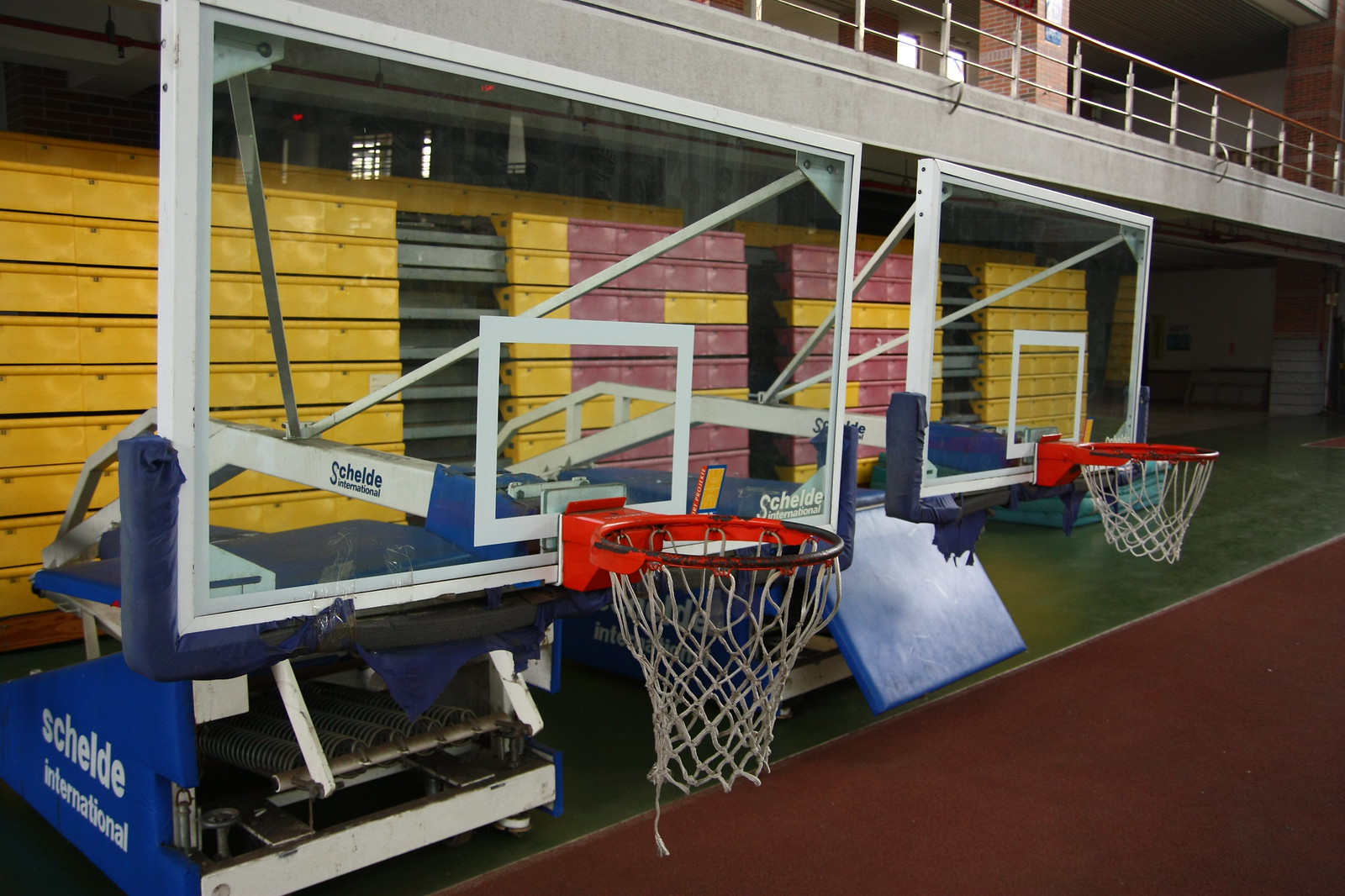The photograph depicts a gymnasium featuring two basketball hoops situated in the foreground. These hoops are not extended upright but are instead positioned close to the floor. They showcase glass backboards, each with a white square at the center and a white frame surrounding it. The rims, which once were orange, now display significant wear with black markings, and the originally white nets appear dingy gray with some frayed strings. Both basketball hoops are supported by blue platforms that bear the name "S-C-H-E-L-D-E International" in white lettering.

Behind the hoops is a wall lined with folded bleachers, predominantly yellow with some maroon sections. Above these bleachers, there is a second-floor level marked by a metal platform with a tan railing, providing a view of the gymnasium below. The gym floor consists of a green laminate slab, likely over concrete, with sections of red carpeting scattered across it. The entire setting conveys a sense of wear and use, giving the gym a rugged and functional appearance.